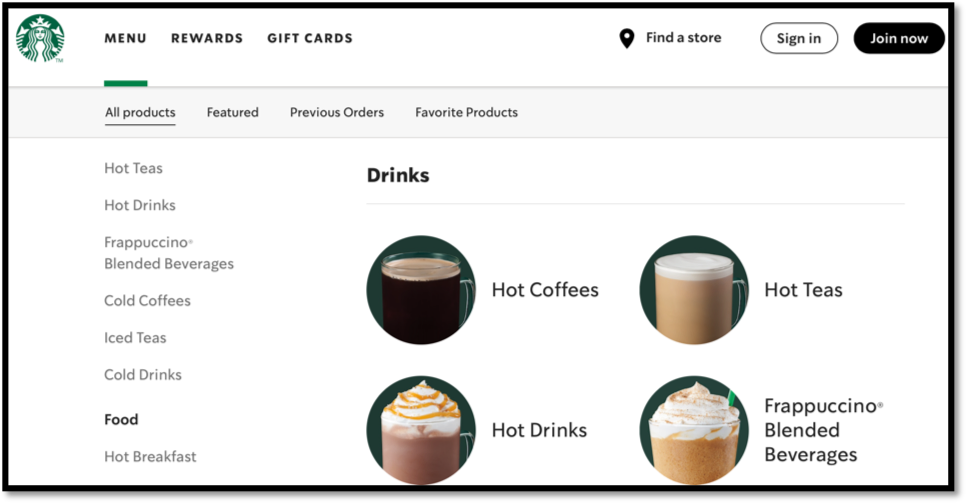The image displays a section of the Starbucks website with a clean, white background outlined by a thin black border. At the top, there's a small circular icon with a green background featuring the iconic Starbucks logo. Adjacent to this logo are the navigational items "Menu," "Rewards," and "Gift Cards," all in bold, dark black text. Further along the navigation bar, there are options for "Find a Store," "Sign In," and "Join Now." The "Sign In" button has a white background with black text, while the "Join Now" button is styled inversely with a black background and white text.

Below the navigation bar is a green separator line followed by a light gray banner. This banner contains the text "All Products," which is underlined, alongside options for "Featured," "Previous Orders," and "Favorite Products." Beneath this banner on the white background, various product categories are listed: "Hot Teas," "Hot Drinks," "Frappuccino Blended Beverages," "Cold Coffees," "Iced Teas," "Cold Drinks," "Food," and "Hot Breakfast," with the "Food" category highlighted in darker print.

Further down, a series of images depict different drink categories. These categories include "Hot Coffees," "Hot Teas," "Hot Drinks," "Frappuccinos," and "Blended Beverages," with each image placed within a circular frame next to its corresponding description.